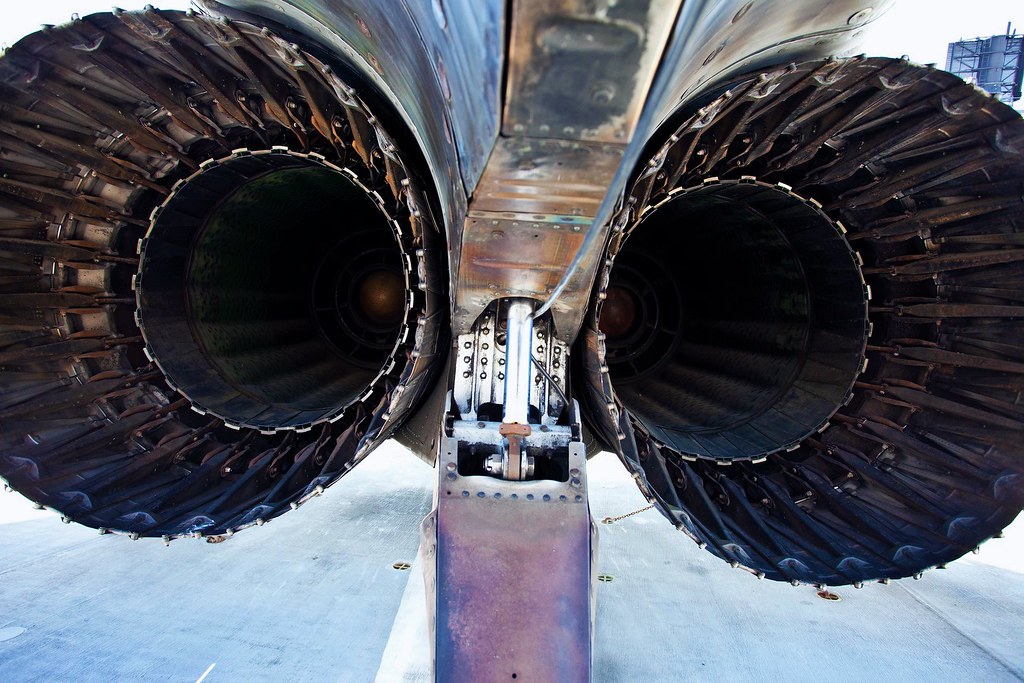This photograph captures a detailed close-up of the rear section of a large, metallic aircraft, most likely a fighter jet, although there are elements that some might mistake for a large rocket. The image dives deep into the intricacies of the machinery, highlighting two large conical structures on either side that resemble jet turbines or engine housings, complemented by a ribbed, coffee filter-like design. The metallic sheen and riveting details from the aircraft's construction are clearly visible, giving a tactile sense to the image. The central part of the photograph showcases an array of gears and levers, likely used to lift a wheel or another component of the plane, hovering above a tarmac with a visible white stripe. In the background, one can faintly discern the reflection of the photographer against the dark metallic surfaces. The machinery's complexity, with its bolts, wires, and moving parts, suggests a mechanism akin to the intricate workings of a jet engine, opening and closing like the iris of an eye.